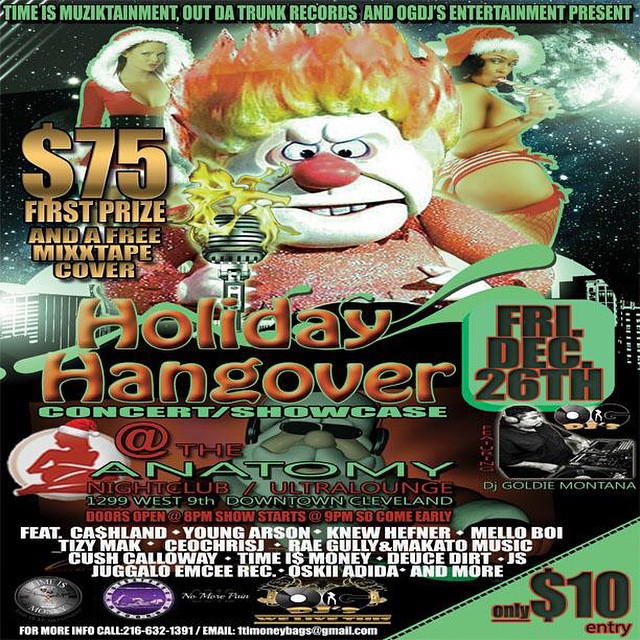The image is a colorful advertisement poster for a music event titled "Holiday Hangover Concert/Showcase." Dominated by green, orange, yellow, and red hues, the poster features a striking central image of a clown-like figure with a white face, red nose, and flaming hair, holding a microphone. Flanking this figure are two women dressed in sexy Santa suits. The event takes place at The Anatomy Nightclub Ultra Lounge in downtown Cleveland, with doors opening at 8:00 PM and the show starting at 9:00 PM. 

Key details include a $75 first prize and a free mixtape cover, prominently advertised. The event is set for Friday, December 26th. It’s hosted by DJ Goldie Montana. The poster also lists a myriad of performers, including Cashland, Young Arson, Canoe Hefner, Mellow Boji, Tizzy Mark, Ray Really, Cash Calloway, Time is Money, D-Tuck, Dirt, JS, Jugga, G-Lope, and more. Entry to the event costs $10. The hosting labels are Music Attainment, Out to Trunk Records, and OG DJs Entertainment.